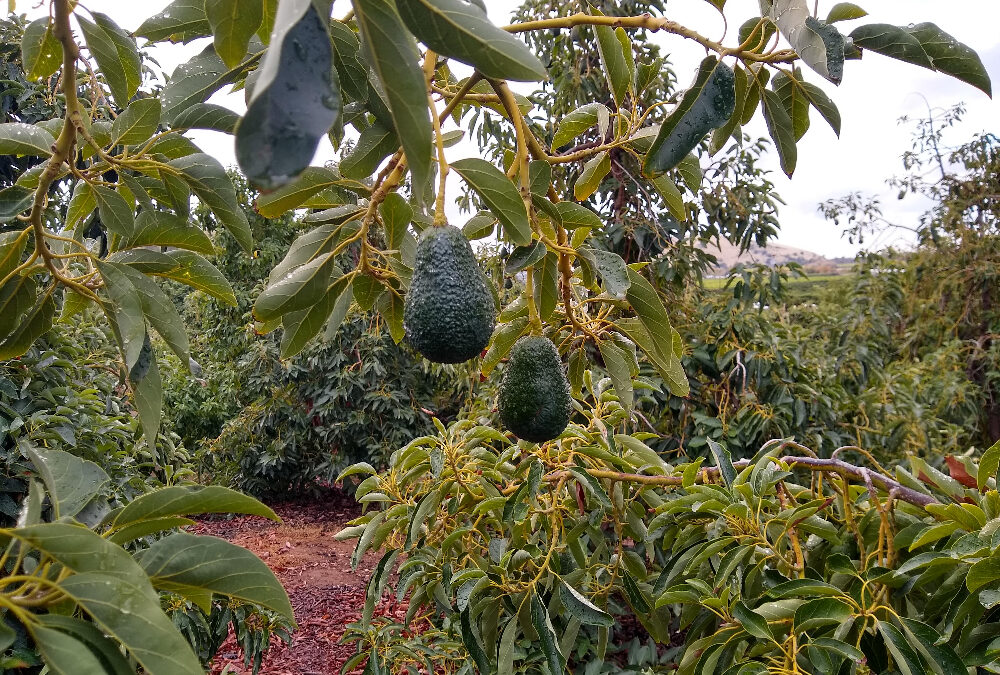This image captures a lush, vibrant garden or field area with a foreground dominated by a brown and red clay-like pathway. On either side of the path, dense green vegetation thrives, featuring a mix of thick leaves and plants. The center of the photo highlights two prominent dark green, pear-shaped avocados hanging from brown branches, with water drops glistening on the surrounding foliage. Behind this focal point, the background reveals a blend of greenery and taller trees, with a stark white, cloudy sky above. To the far right, a hint of a mountainous region adds depth to the scene. The avocados appear larger than normal, about 10 to 12 inches long, adding an intriguing focal point to the lush landscape.